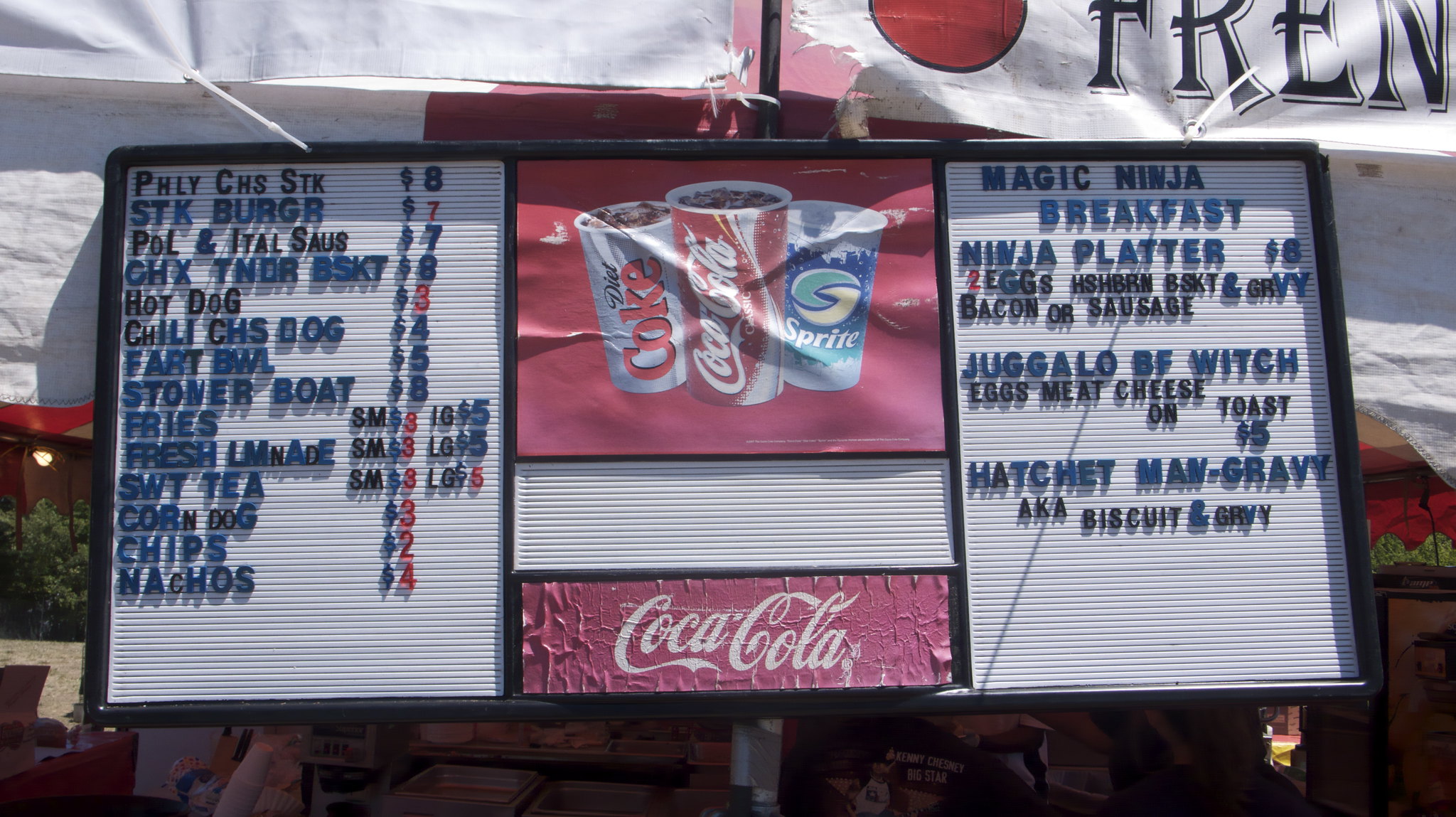In this image, we see a photo of a food stand's menu sign. At the top right corner of the sign, partially obscured, is what appears to be the establishment's name, showing half of a red circle and a few letters that might spell "FREN," though the rest is cut off. The main sign in the center features images of various beverages, including Diet Coke, Coca-Cola, and Sprite, set against a red background with the Coca-Cola logo at the bottom.

On the left side of the sign, the menu items are listed, offering a variety of foods such as Philly Cheese Steaks, Steak Burgers, Italian Sausages, Impola Sausages, Chicken Tender Baskets, Hot Dogs, Chili Cheese Dogs, a unique item named the Fart Bowl, a Stoner Boat, Fries, Fresh Lemonade, Sweet Tea, Corn Dogs, Chips, and Nachos.

The right side of the sign advertises "Magic Ninja" breakfast options. The breakfast menu includes a Breakfast Platter with eggs, hash brown baskets and gravy, and a choice of bacon or sausage. They also offer a "Juggalo B.F. Witch," which is a sandwich with eggs, meat, and cheese on toast, as well as the "Hatchet Man Gravy," which is biscuits and gravy.